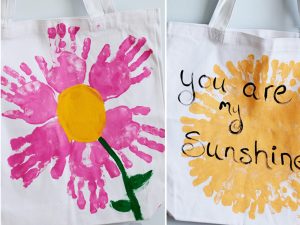The image features two distinct panels set against a white background, each depicting a white linen canvas bag adorned with hand-painted designs. The left panel showcases a grocery or storage bag embellished with a charming, handmade flower. The flower's petals are created from six child-like handprints arranged in a circle, painted in pink and purple hues. At the flower's heart lies a yellow, circular center, from which a green stem descends diagonally toward the lower right corner, adorned with two small green leaves.

On the right panel, another white linen bag presents a radiant depiction of a sun. This design features a large, orange-yellow circle, artistically sponged to give a textured appearance, representing the sun with radiating rays. Above this vibrant sun, the phrase "You Are My Sunshine" is inscribed in bold black text, adding a heartfelt touch to the sunny illustration. Both panels capture the essence of simple yet expressive child-like artwork, merging vibrant colors and meaningful messages.